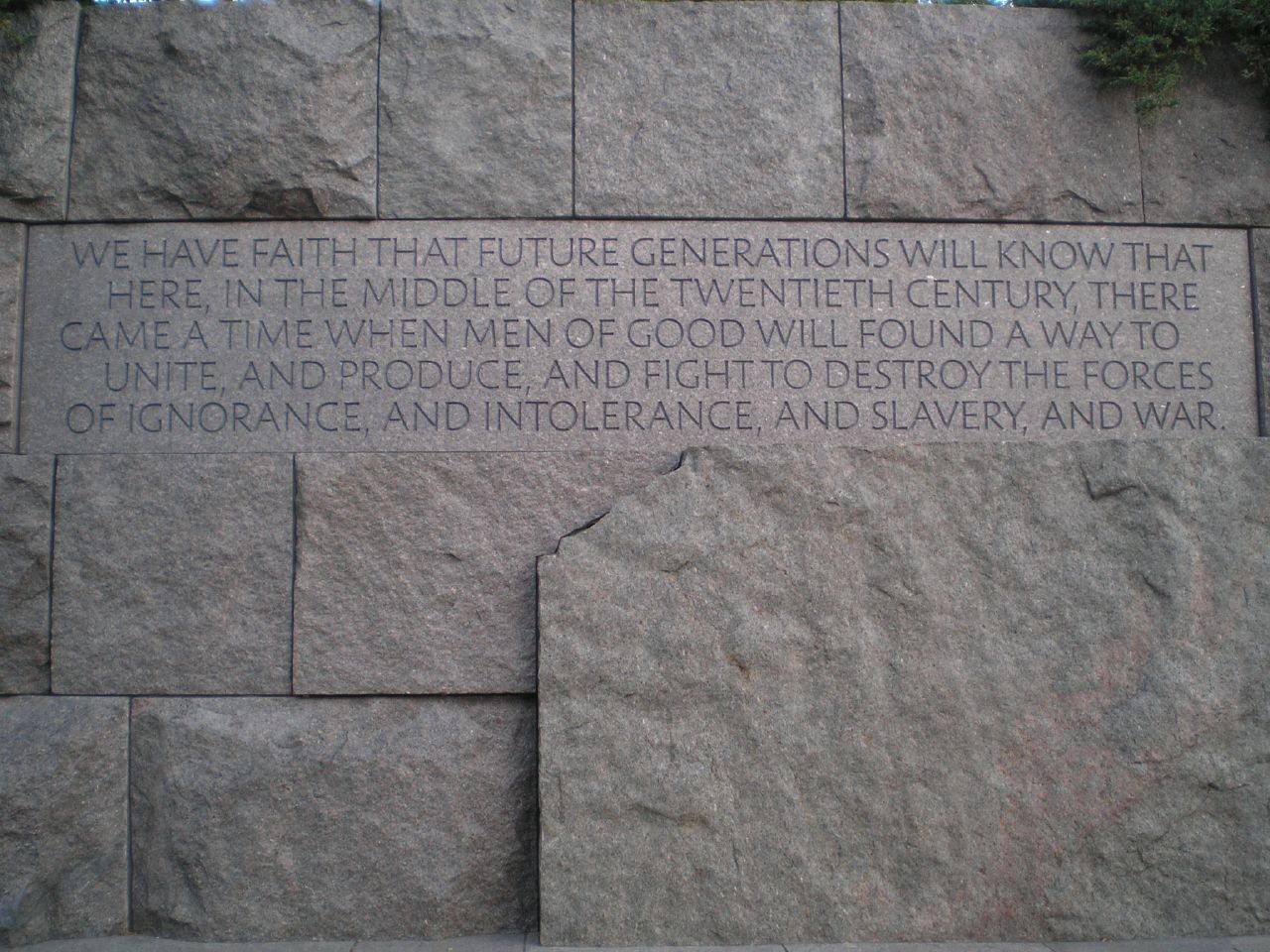The image depicts a section of a memorial or monument made of medium gray concrete or stone bricks, arranged in a rectangular and square pattern. It features a wide rectangular engraving located on the second row from the top. The inscription is in all capital letters and reads, "We have faith that future generations will know that here in the middle of the 20th century, there came a time when men of goodwill found a way to unite and produce and fight to destroy the forces of ignorance and intolerance and slavery and war." The surface of the bricks appears smooth yet bumpy, adding texture to the structure. In the top right corner of the image, a portion of a green bush or tree is visible, providing a natural contrast to the gray stone.